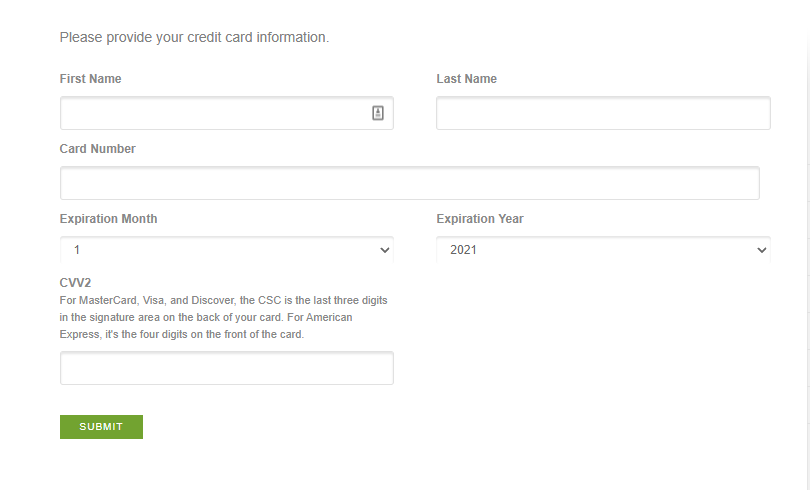The image shows a credit card information form from a website, presented on a white background with a subtle gray border along the right-hand side. At the top left corner, there is a heading asking users to "Please provide your credit card information." 

Below this heading, the form is organized into several fields with bolder gray labels. The first field is labeled "First Name" and has an input space immediately below it. To the right of this, there is a field labeled "Last Name" with a corresponding input space beneath it.

Next, the form requires the "Card Number" with an input slot directly below this label. Following this are fields for the card's expiry details: "Expiration Month," which features a drop-down menu currently displaying the number one, and "Expiration Year," which also has a drop-down menu set to the year 2021.

The last section of the form is dedicated to the card's security code. It prompts for the "CVV2 for MasterCard, Visa, and Discover," noting that this code consists of the last three digits found in the signature area on the back of the card. For American Express cards, users are instructed to input the "four digits on the front of the card." There is a blank area below this explanation for entering the CVV2 code.

At the bottom of the form, a green button with white text is labeled "Submit."